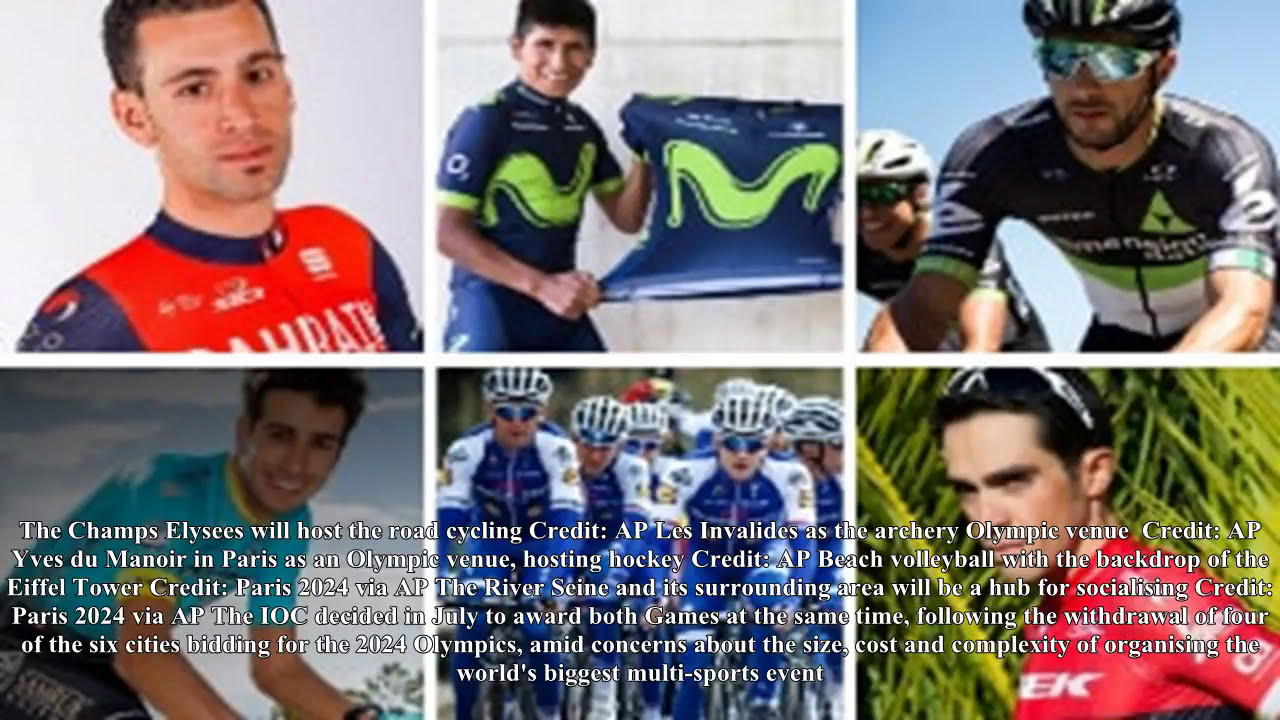The image is a collage of six photographs featuring competitive cyclists, arranged in two rows of three. The top left photograph shows a clean-shaven cyclist in his 20s or 30s, wearing a red jersey with blue sleeves, although the text on the jersey is not legible. The top center image features another cyclist clad in a blue uniform with a green wave design, holding up a matching jersey and smiling. The top right photograph depicts a cyclist on his bike, wearing reflective shades and a helmet, his jersey adorned with black, green, and white stripes; another cyclist's helmet is partly visible on the left edge of this photo. 

The bottom left image captures a darkened photo of a clean-shaven cyclist in a light teal jersey, leaning forward as if riding. The bottom center picture displays a 'peloton,' a tightly-knit group of at least ten cyclists, all in blue jerseys with white-shouldered sleeves. Lastly, the bottom right photo presents a cyclist in a red jersey with white text, standing in front of palm tree fronds, with shades resting atop his head. There is a broad caption running across the bottom images, providing credits to the photographers and containing text about the Paris 2024 Olympics, though much of the detailed captioning is obscured by the colorful background of the images.